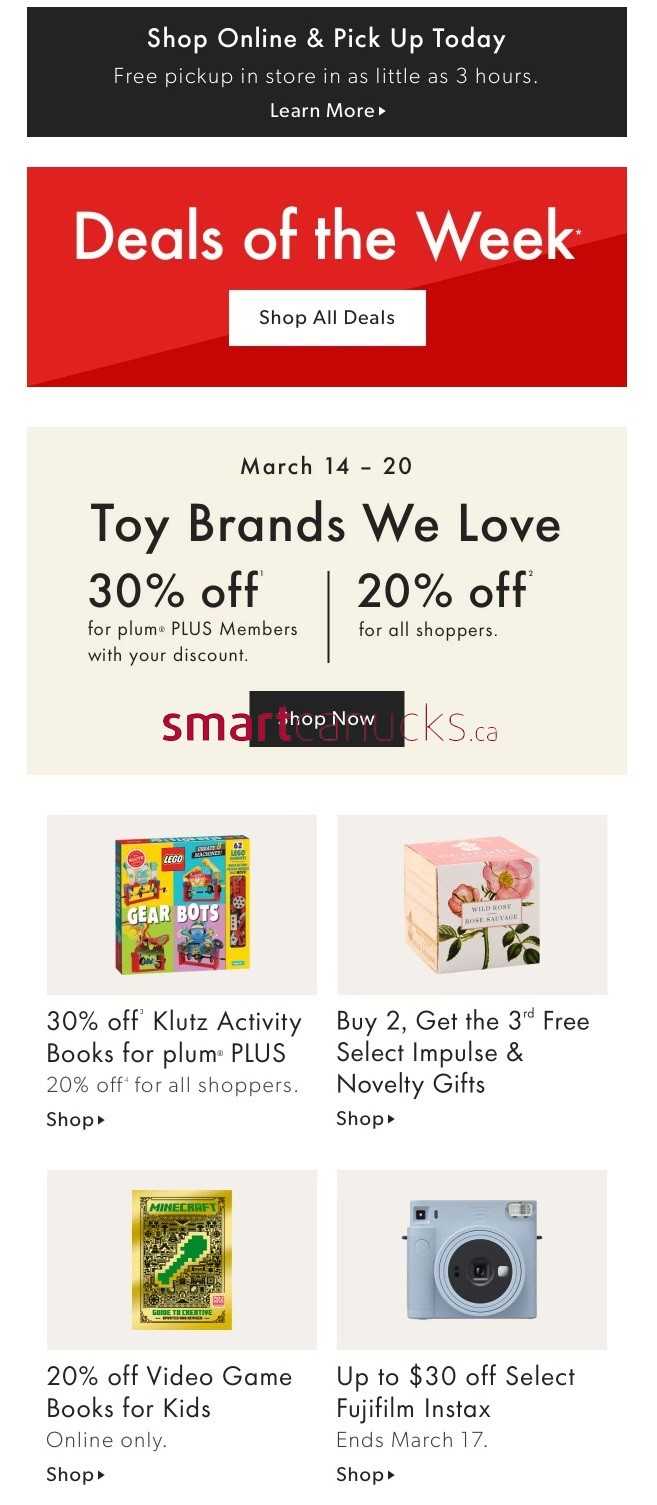The image is a screenshot from a store's "Deals of the Week" promotional page. At the top of the screenshot, a black bar with white text reads, "Shop Online and Pick Up Today," with a subtext below stating, "Free Pickup in Store in as Little as 3 Hours." Adjacent to this text is a pull-down menu labeled "Learn More."

Below this section is a prominent red box with white text indicating "Deals of the Week." Within the red bar lies a clickable white link titled "Shop All Deals."

The main section of the image details the specific weekly deals, valid from March 14th to March 20th. It highlights that toy brands are available at a 30% discount for Plum Plus members and a 20% discount for all other shoppers, with a "Shop Now" link provided for more details.

The deals feature four highlighted products:
1. In the upper right quadrant, there's a deal for Klutz activity books at 30% off for Plum Plus members and 20% off for all shoppers. An accompanying image showcases the books.
2. Next to it, there's an offer for select impulse and novelty gifts available at a "Buy Two, Get Three Free" deal.
3. Below the Klutz activity books deal, a promotion offers a 20% discount on video game books for kids, with an image of one such book above the text.
4. In the bottom left section, there's a deal offering up to $30 off select Fujifilm Instax cameras, accompanied by an image of one of the cameras.

Overall, the screenshot effectively presents the store’s enticing weekly deals, complete with visually appealing product images and clear discount information.